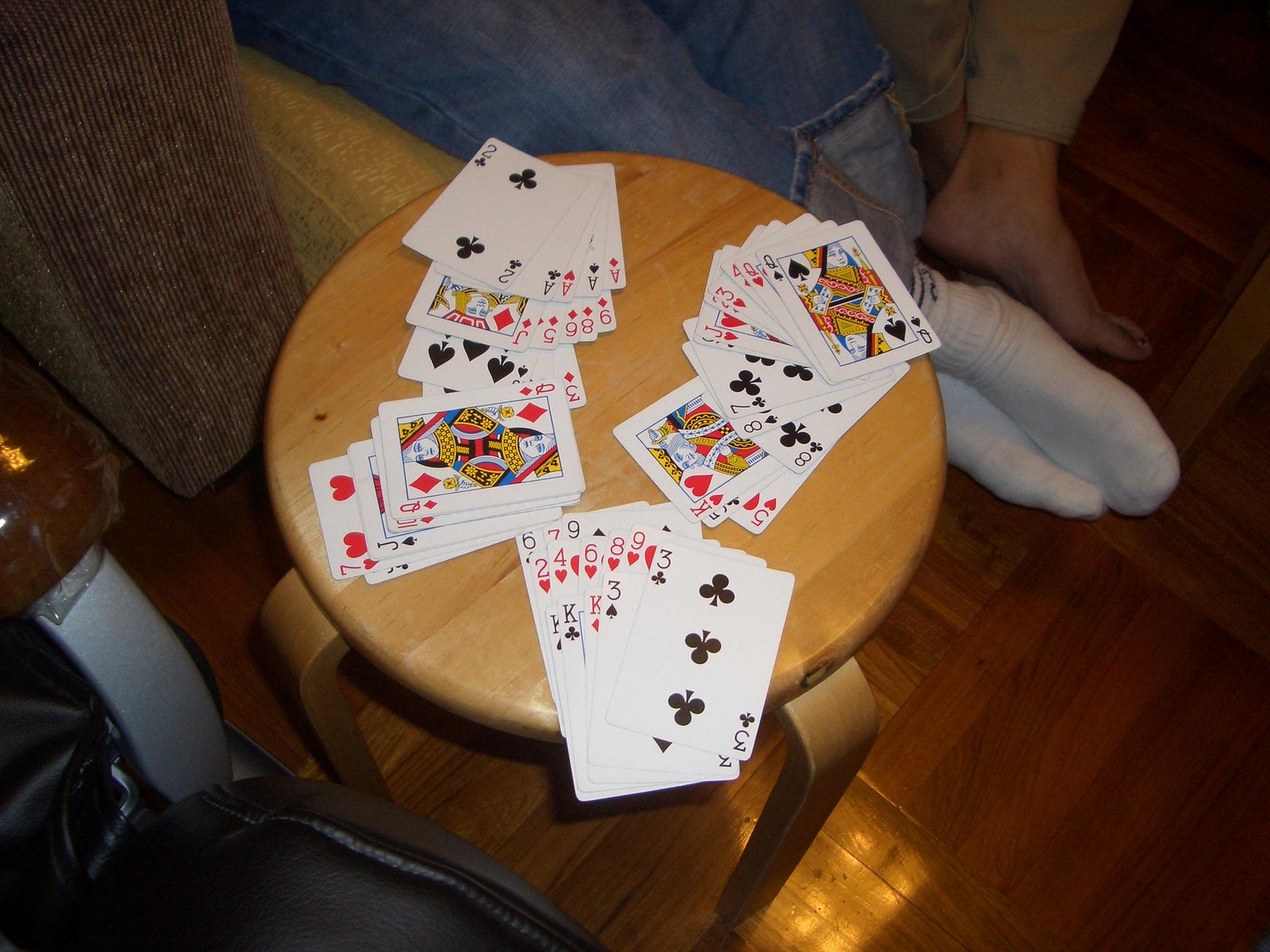The image features a light brown wooden end table, prominently positioned with its four legs visible. Atop this small table are four distinct piles of playing cards, reminiscent of a poker game. The bottom-most pile reveals the three of clubs, while the pile to its left is topped by the red queen of diamonds. Above and to the right of this pile lies another with the two of clubs visible on top. The final pile, positioned to the far right, is capped with the black queen of spades. Surrounding the table, to the upper left, stands a brown and yellow patterned couch. Seated upon this couch are two visible pairs of legs - one draped in blue denim jeans with white socks, and the other in tan corduroy pants, featuring bare feet of a pale complexion. Adjacent to the end table on the bottom left corner is a brown leather office chair. The scene is completed by a clean, light brown laminated wooden floor that extends across the room.